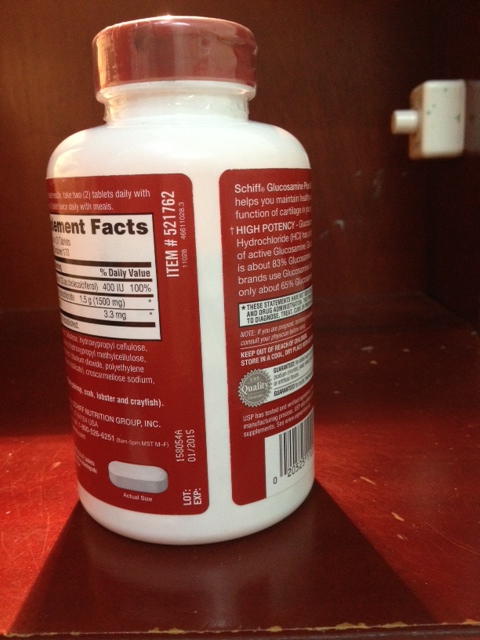A white bottle containing capsule medicine or vitamins is prominently displayed on a cherry wood desk, which exhibits noticeable scratches and patches where the wood is scraped away. The bottle features a red lid that is sealed with clear plastic wrap and a matching red label. The label includes an image of the actual white capsule, marked with "actual size," and partially visible nutrition facts. The bottle itself shows item number 521762 and the word "quality," with a note indicating that the statements are not approved by the USDA. Slightly turned, the bottle casts a shadow on the desk. In the upper right corner of the image, a white, square-shaped box with a protruding circular button is visible. Behind the desk, there is a matching cherry wood wall or back panel.